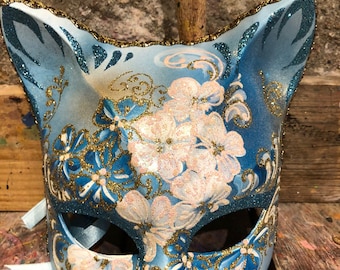The image is a close-up, bright, and highly detailed color photograph of a mask that resembles a cat's head, complete with prominent cat ears at the top corners. The mask exhibits a striking blue and white color scheme, adorned with a floral pattern featuring roses and highlighted areas accented by gold and blue glitter that make the surface almost appear computer-generated due to the sparkle effect. The mask is positioned against a background comprising gray stone blocks with a wooden board spanning the center, possibly an old wooden tabletop. The photograph only shows the upper portion of the mask from the eyes up, revealing black eye holes while the rest of the mask is cut off, emphasizing just the intricate upper design and texture of the item.